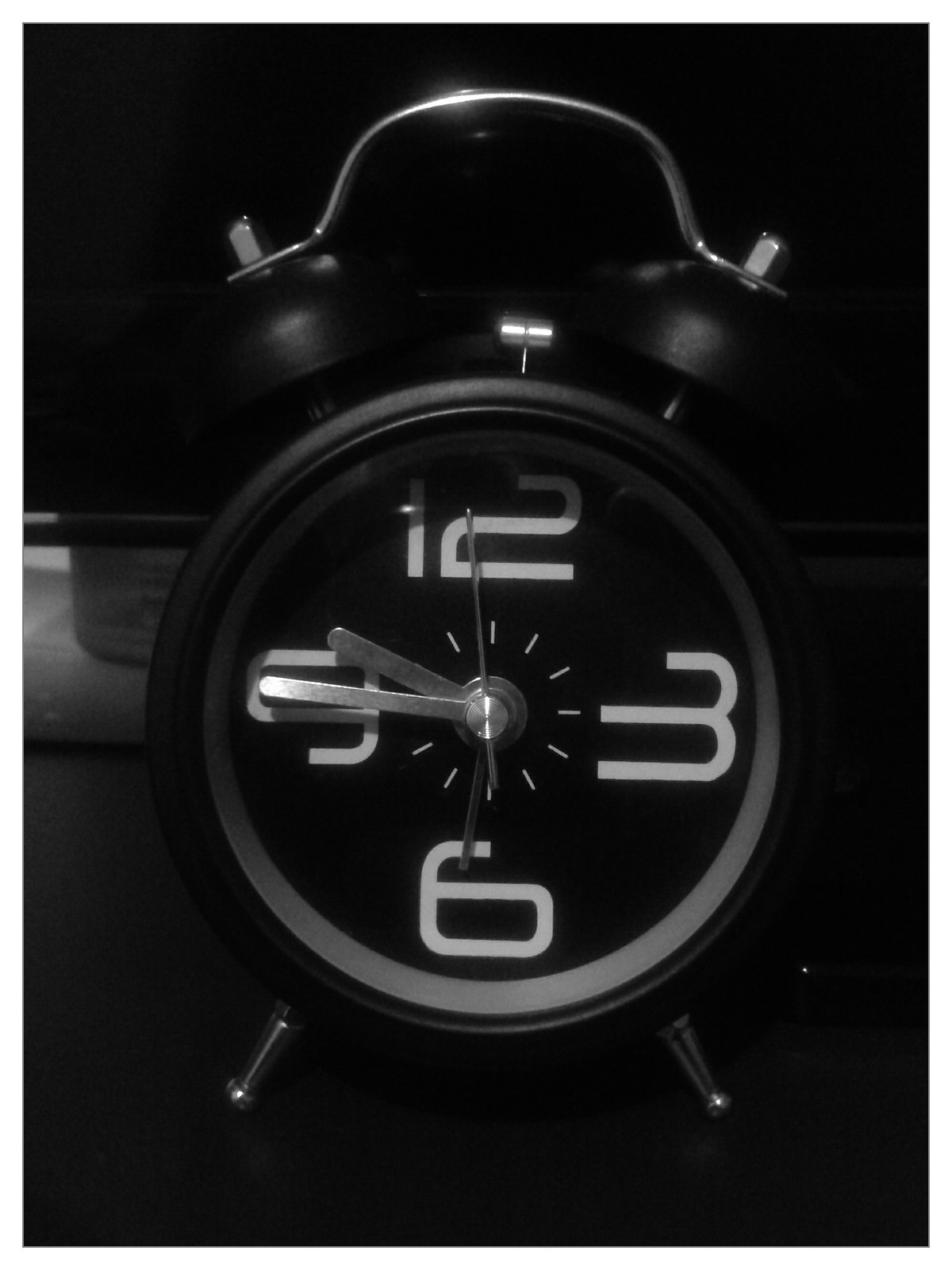This black-and-white photograph captures a close-up of a small, vintage-style alarm clock, set against a nearly pitch-black background, lending a dramatic contrast that makes the object pop. The alarm clock is sleek and black with a round face, supported by silver legs ending in small decorative orbs. Perched atop the clock is a classic old-school analog alarm mechanism, featuring two substantial bells on either side, connected by a silver hammer designed to strike them for the alarm sound. The clock face displays only three numerals—12, 3, and 6—in a large, retro-stylized font, which adds to the nostalgic aesthetic. The time appears to be approximately 9:45, though the exact minute is difficult to discern. The expertly lit scene and the detailed design of the clock evoke a sense of timeless elegance and functionality.